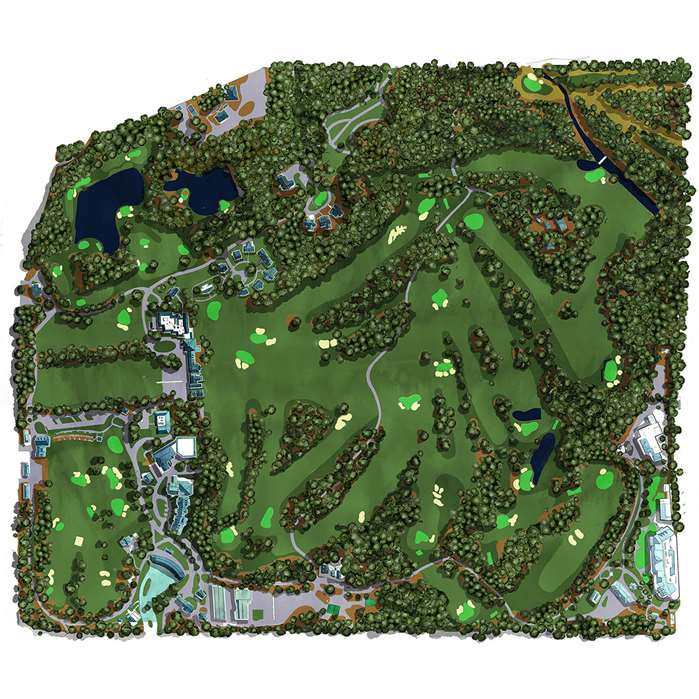This detailed aerial illustration of a lush golf course is densely populated with greenery, featuring a network of trees that dominate the upper region and borders of the image, interspersed with clearings revealing the meticulously designed course. The image highlights multiple putting greens in various light green shapes, surrounded by strategically placed white sand traps. In the top right, a river or stream meanders through the trees toward a hole, adding a scenic element. In the top left, the course is adjacent to two large ponds and a building speculated to be part of a country club. More buildings can be seen in the bottom left, including dark blue and cyan roofs, flanking a winding gray concrete path, and a large parking lot housing long olive green structures. The bottom right also contains additional buildings. The course is rich in diverse topographical features, with ponds of varying shapes—including a horseshoe and fish-shaped pond—emphasizing its complexity and aesthetic appeal.